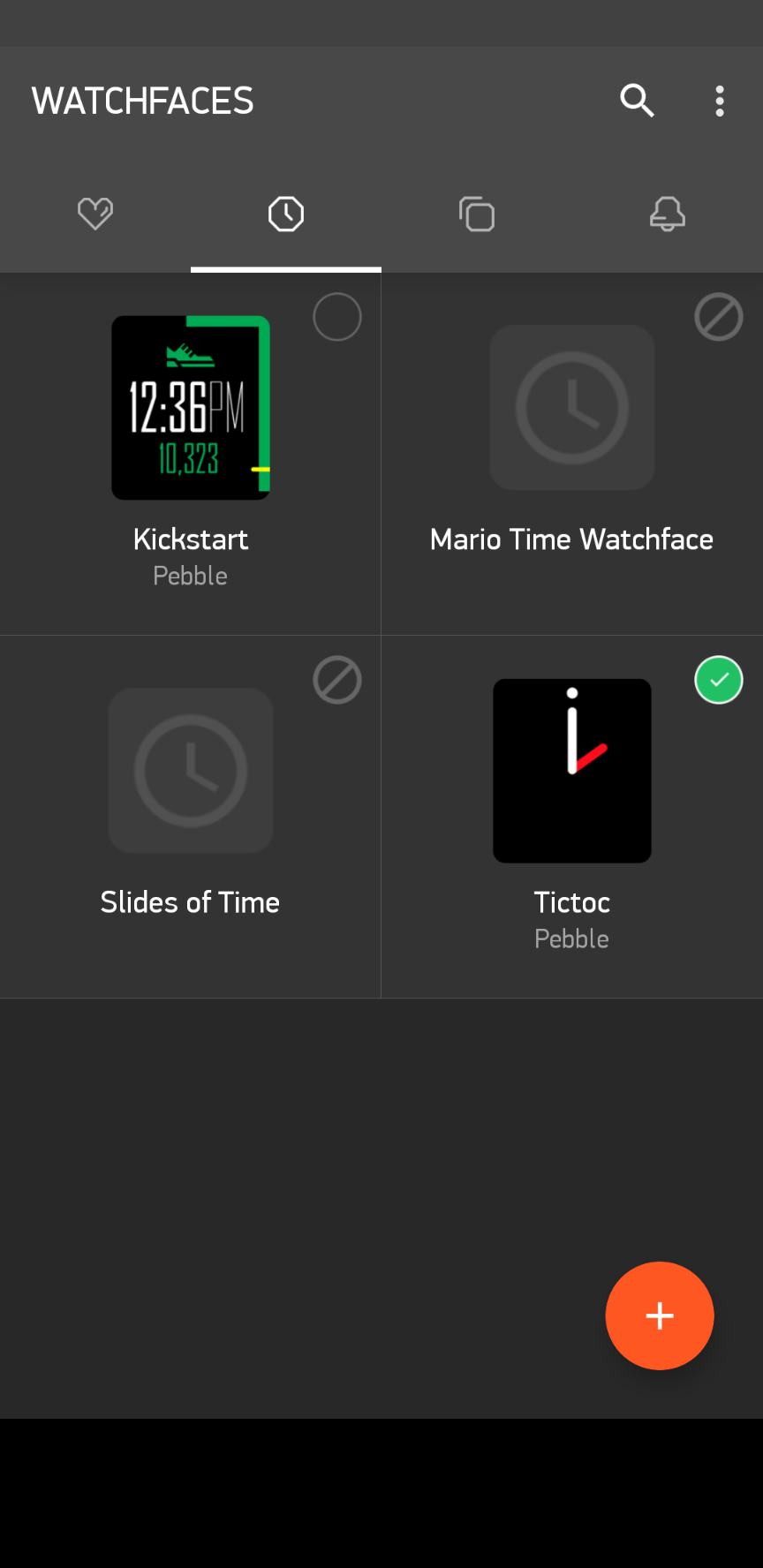This image is a screenshot from an unspecified web page with a dark gray background. At the top of the page, the text "WATCHFACES" is prominently displayed in uppercase white letters. On the top right corner, there are two icons: a magnifying glass and a set of three vertical dots.

Beneath this, there are four icons aligned horizontally: a heart, a clock face (which is currently selected), an overlapping squares icon, and a bell. Following these icons, on the left side, there is a black icon with a green border that starts from the middle of the top edge and extends down the right side. This icon features a green drawing of a shoe. Below this icon, the text "12:36 PM" is displayed in white letters, and directly underneath it, the number "10,323" is shown in green. Below these details, the text "Kickstart Pebble" appears.

To the right of this, there is a gray square featuring a gray clock face, labeled "Mario Time Watch Face." Further down in the following row, there is another gray square with the same clock face icon, labeled "Slides of Time."

Finally, there is a black icon with a minimalist design: a lowercase "i" with a red diagonal line emanating from its bottom right, forming an abstract clock face. This icon is also selected and is labeled "tictoc pebble." At the very bottom of the image, there is an orange circle with a white plus sign centered within it.